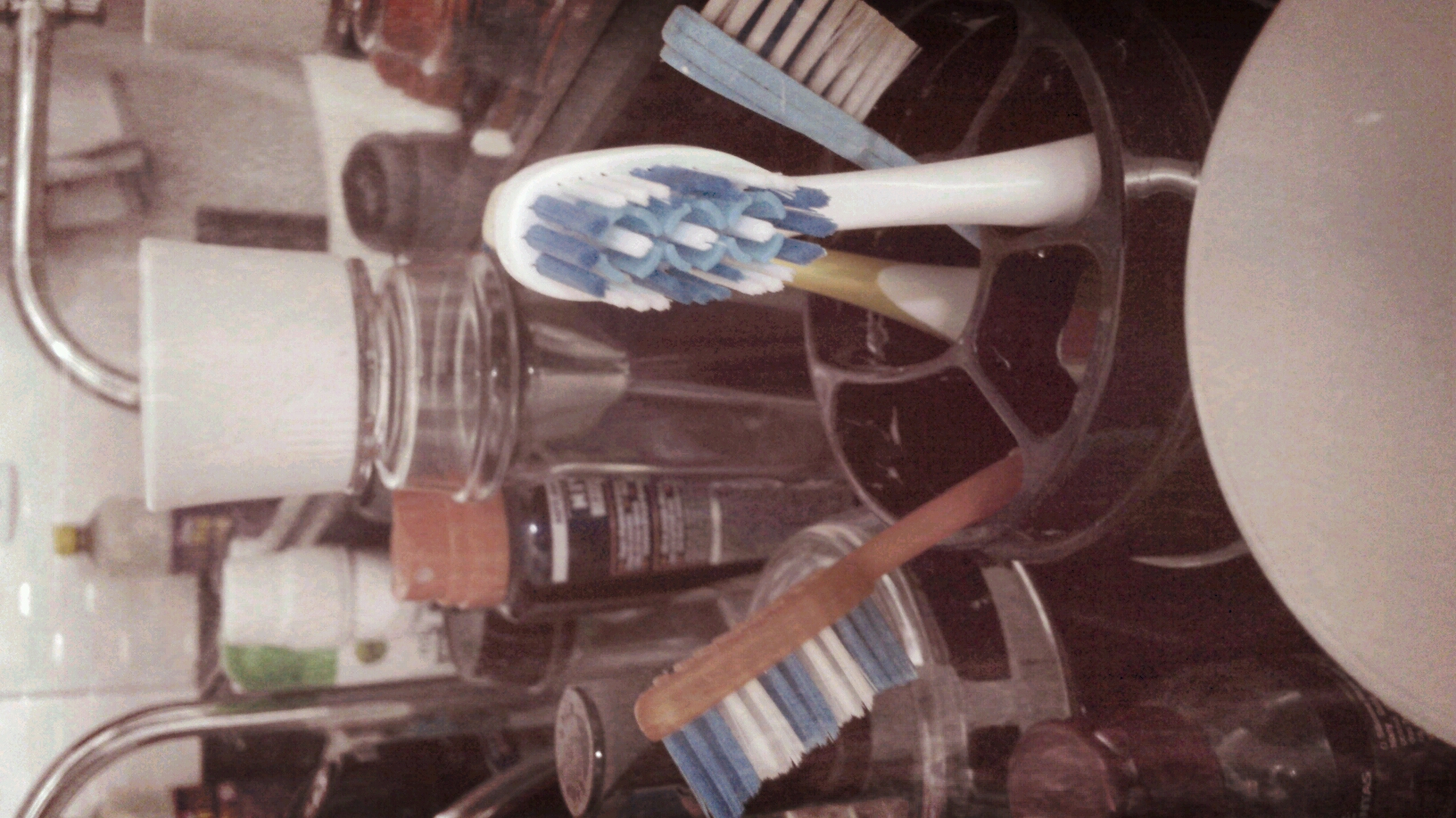The image is a close-up shot of a sink area that features predominantly cleaning items. At the forefront, there is a toothbrush holder cup containing four toothbrushes: one white with blue and white bristles, one red on the left with blue and white bristles, one yellow and white, and one light blue with white bristles. Behind the toothbrushes, there's a clear bottle with a white cap, although it does not appear to contain any visible content. Additionally, there are various other bottles including a brown bottle with a tan cap, a white bottle with a green cap, and another white bottle with a white cap, which might be shaving cream. A glass bowl is placed in front of the toothbrushes, and the background features the sink's faucet. The setting suggests this is possibly a bathroom, but the presence of numerous cleaning chemicals and containers adds ambiguity, hinting it might also be a garage or workshop sink used for cleaning tools or parts.